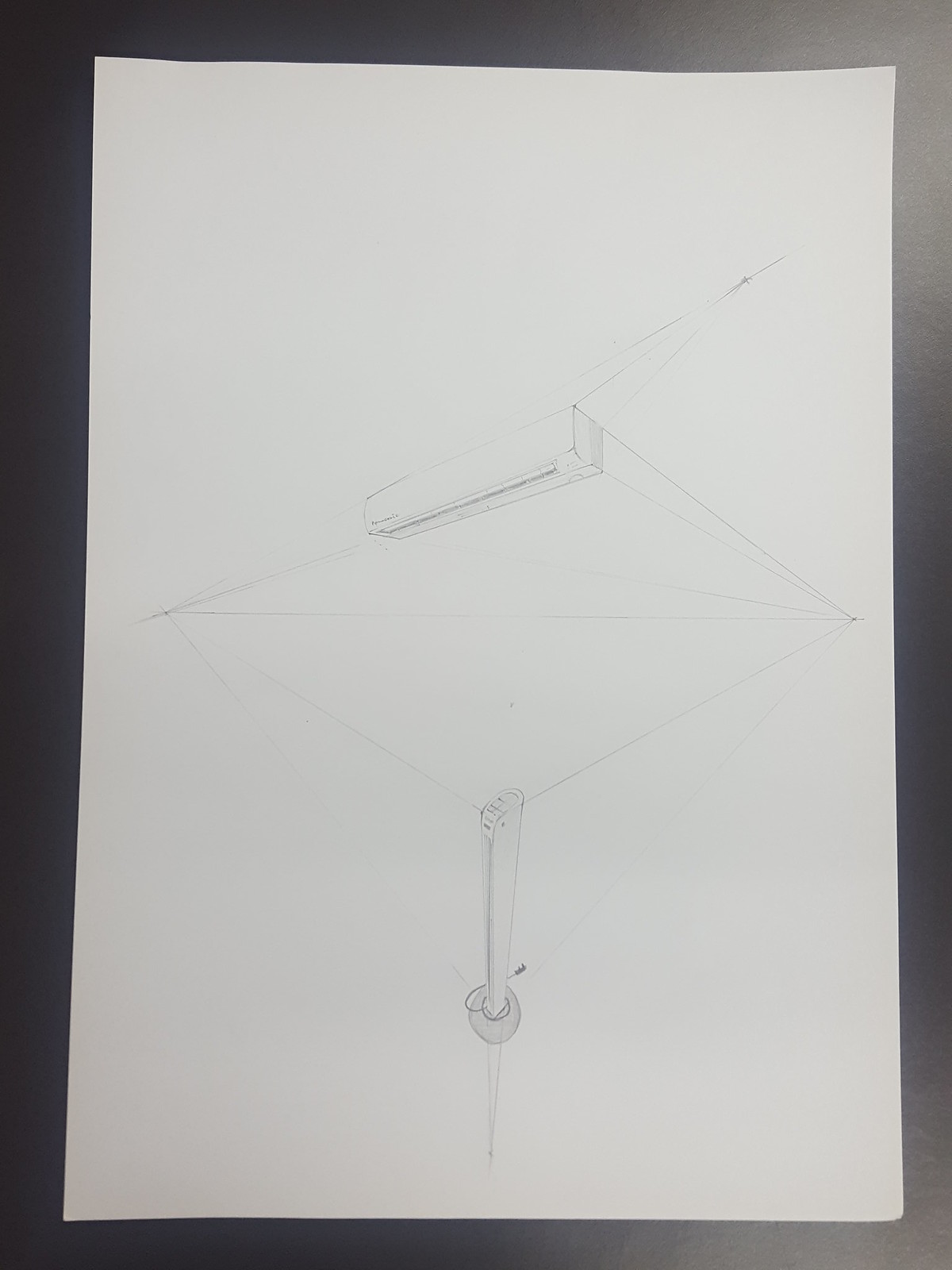The image features a black-bordered frame enclosing a white piece of paper. On this paper, there are exceedingly faint line drawings, sketching what appears to be a structural diagram for a potential build project. One segment of the sketch resembles a drawer, while another portion shows what looks like a table leg connected to a corner of the construction. The design seems indicative of a folding table blueprint, especially given the presence of a hinge mechanism that suggests the table might fold up. Despite attempts to enhance visibility through lighting adjustments, the lines remain incredibly faint and difficult to discern.